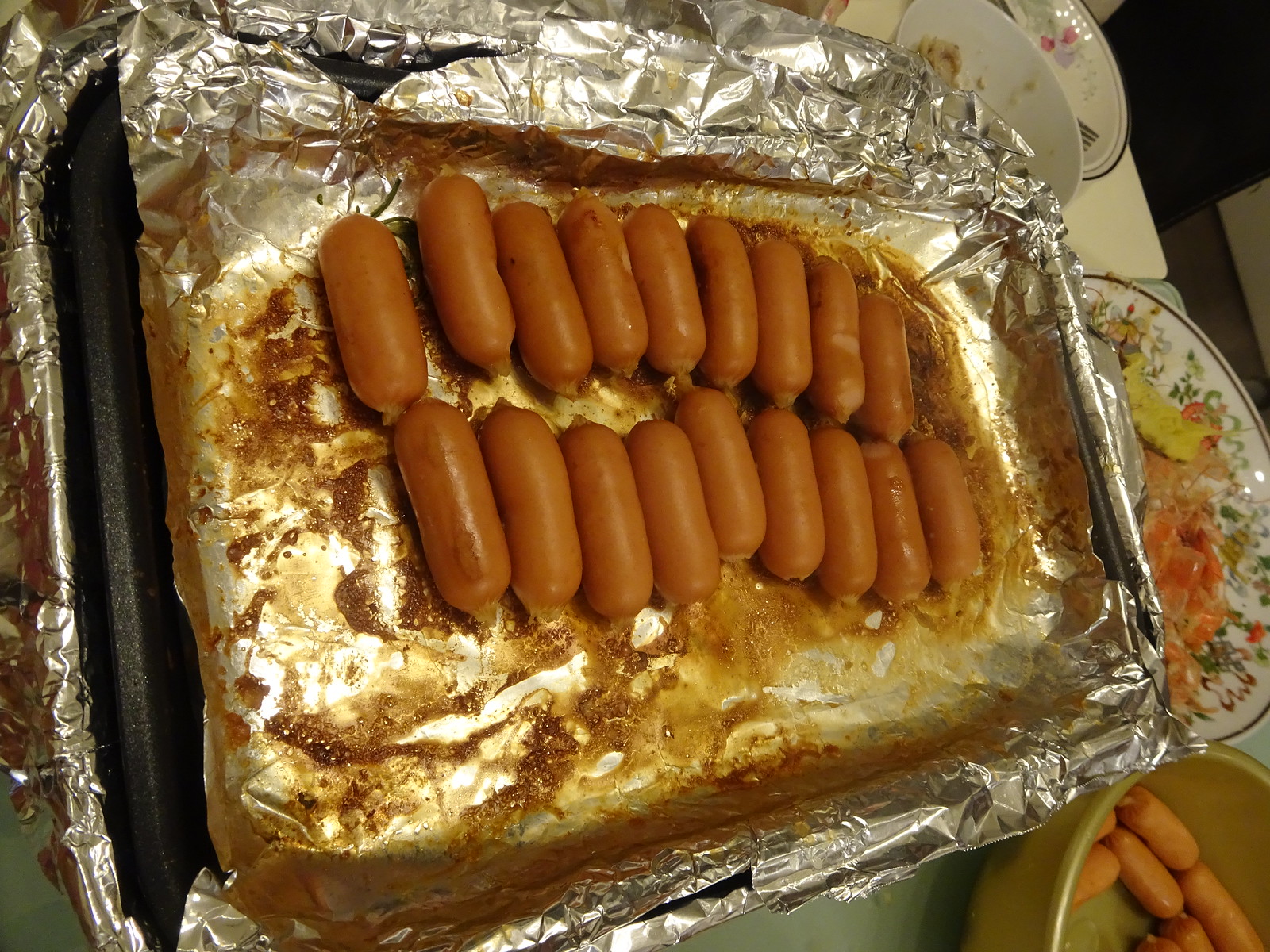In this detailed image, we observe a metal tray lined with aluminum foil, holding approximately 19 small, cooked sausages arranged in two neat rows. Some sausages appear connected by their casings, glistening with grease from the cooking process. This scene suggests a party setting with various finger foods. Nearby, a green bowl contains additional uncooked sausages. Adjacent to these, a ceramic plate adorned with floral designs holds a serving of avocado and shrimp, indicating these items might have already been partially consumed. The background also features scattered dirty bowls and dishes, reinforcing the idea of an ongoing or recently concluded gathering.